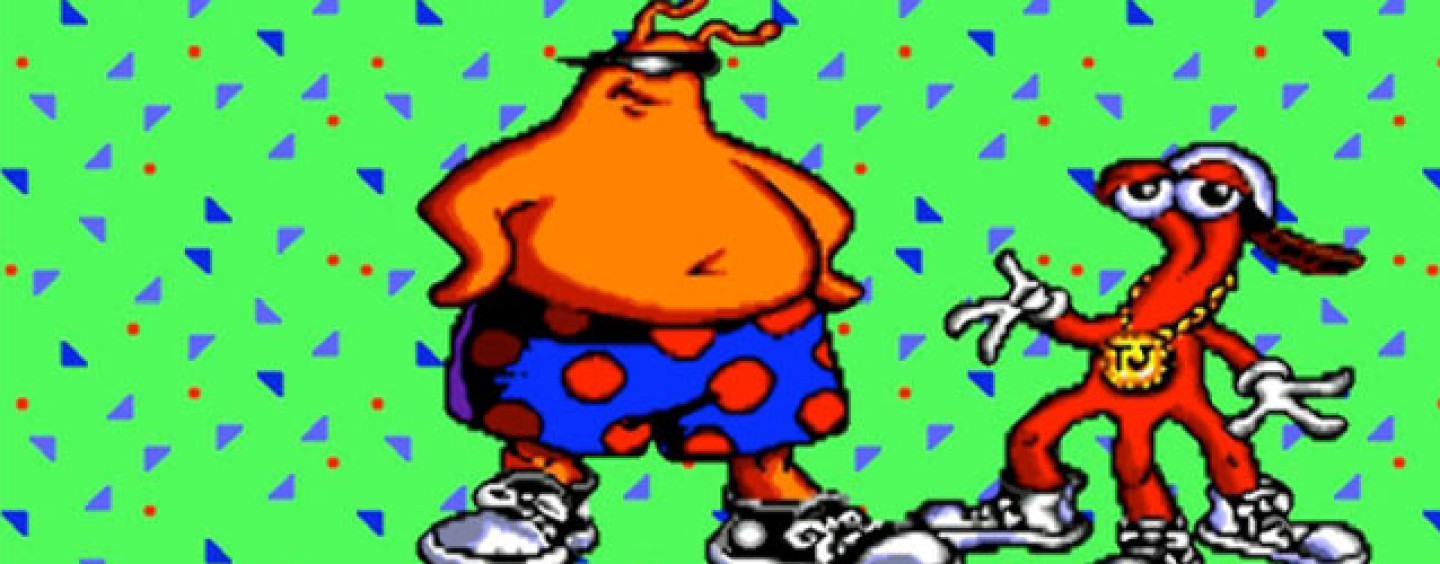This image is a detailed, vibrant graphic from the early 1990s Sega Genesis game ToeJam & Earl. The scene takes place in a rectangular, bright teal green background adorned with small blue, purple, and red geometrical shapes, including triangles and dots. Two distinctive cartoon characters are prominently featured.

On the left side is the larger character, Earl. He is a bright orange, large-bellied creature with squiggly antennae on his head. Earl sports black sunglasses that block out a significant amount of light and wears blue shorts with red polka dots. His shoes are black and white and oversized for his big feet, adding to his quirky appearance.

To the right is ToeJam, an even more alien-looking figure. He is red with a unique three-legged structure, each leg ending in oversized shoes. ToeJam's small eyes sit atop stalk-like appendages, and he wears a baseball cap turned backward on his head. A defining feature is his gold necklace with the initials "TJ," confirming his identity.

Together, these characters against the colorful, geometrically-patterned backdrop encapsulate the whimsical essence of the ToeJam & Earl game.